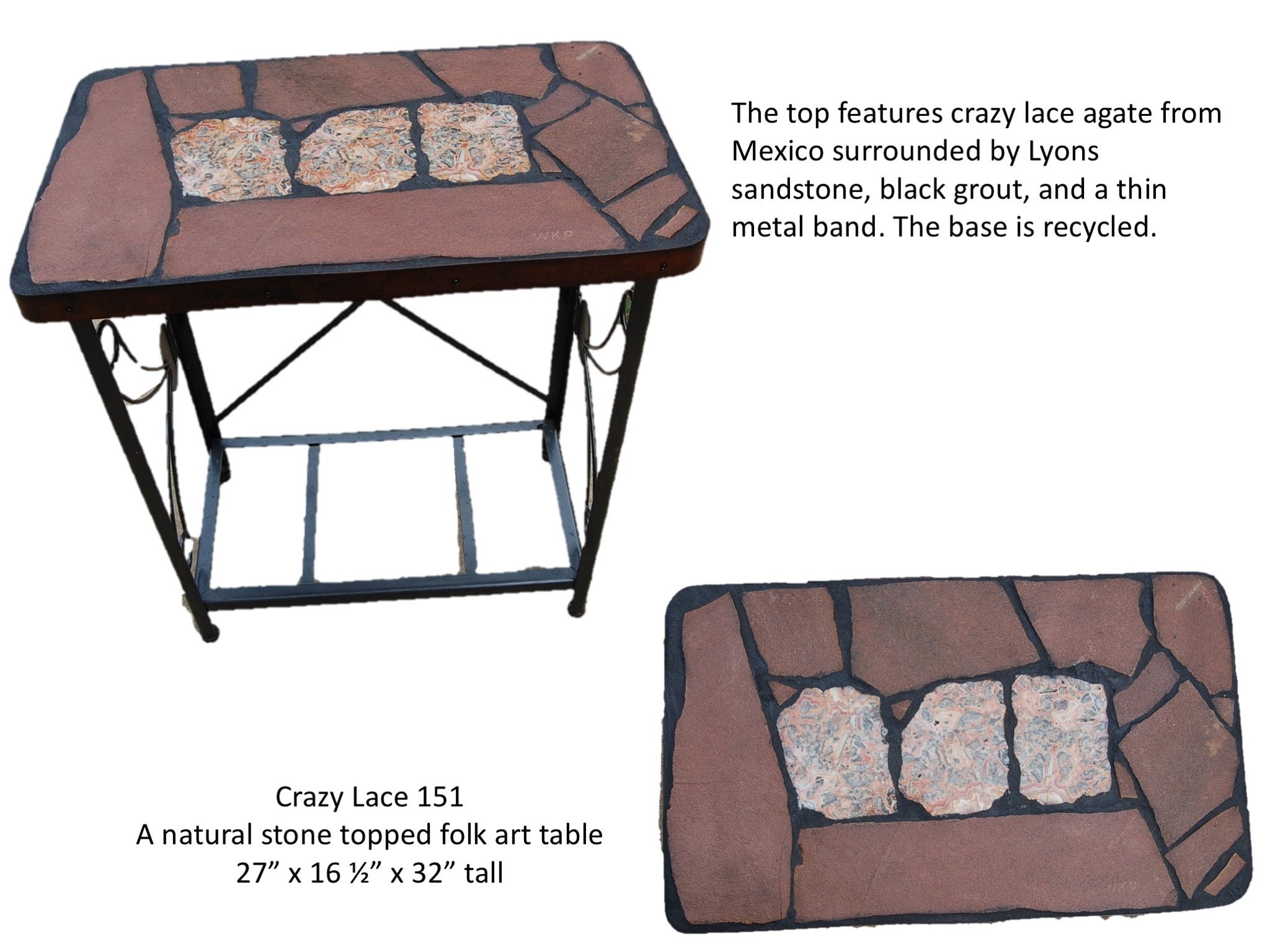The image depicts a unique folk art table prominently featuring two different perspectives. The top-left section showcases a side view of the table, highlighting its black metal legs and frame. Adjacent to this, the caption reads: "Crazy Lace 151, a natural stone-topped folk art table, 27 inches by 16.5 inches by 32 inches tall." The table’s top, prominently visible in the bottom-right section, is crafted from Crazy Lace Agate from Mexico. This stunning agate center, exhibiting yellow and gray tones, is bordered by darker brown stones with black grout in between and encircled by a delicate metal band. The text further clarifies that the table’s solid yet artistic base is made from recycled materials, ensuring both aesthetic appeal and sustainability.